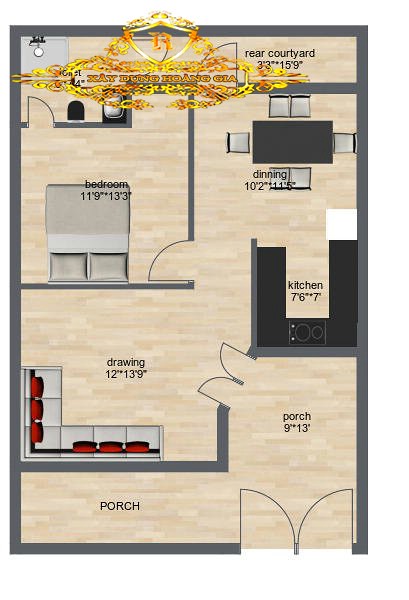A digital blueprint or layout of a house with a gray border outlining its walls. Upon entering from the right corner, there is an inviting porch to the left, extending further as you walk in, measuring 9 feet by 13 feet. An angled door leads into the main living space, labeled as "Drawing 12, 13, 9." This area features seating with red pillows on gray furniture, set against wooden flooring.

Moving upward and to the left, you encounter a bedroom with the bed positioned against the wall. Adjacent to the bedroom is a bathroom equipped with a toilet and a shower. To the right of the bathroom is the kitchen, a compact 7 by 7 feet space designed in a sleek black finish.

Directly in front of the kitchen is the dining room, and to its left, a door opens up to a cozy rear courtyard.